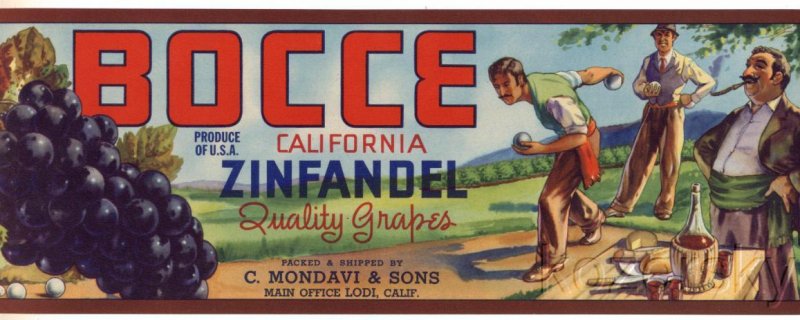This vintage wine advertisement, likely from the 1950s, appears to be designed as a label for a Zinfandel wine bottle. The label, which is wide and horizontally rectangular with brown borders, prominently features the brand name "Bocce" in large red text with a black outline at the top left. Below, smaller red text reads "California," followed by "Zinfandel" in dark blue, and "Quality Grapes" in red cursive. At the bottom, in very small black text, it states, "Packed and Shipped by C. Mondavi and Sons, Main Office, Lodi, California." 

The left side of the label displays an illustration of dark purple grapes with leaves above them. On the right side, the scene depicts three men dressed in older attire, engaging in what appears to be a game of bocce ball. One man, ready to toss the ball, has his arm extended behind him, while another prepares to throw a ball as well. A third man, heavier set with a mustache, is smoking a pipe and stands by the picnic table adorned with a bottle of wine, cheese, and bread. The men in the illustration, with their Italian appearance and the recreational setting, add a rustic and nostalgic touch to this classic wine label.